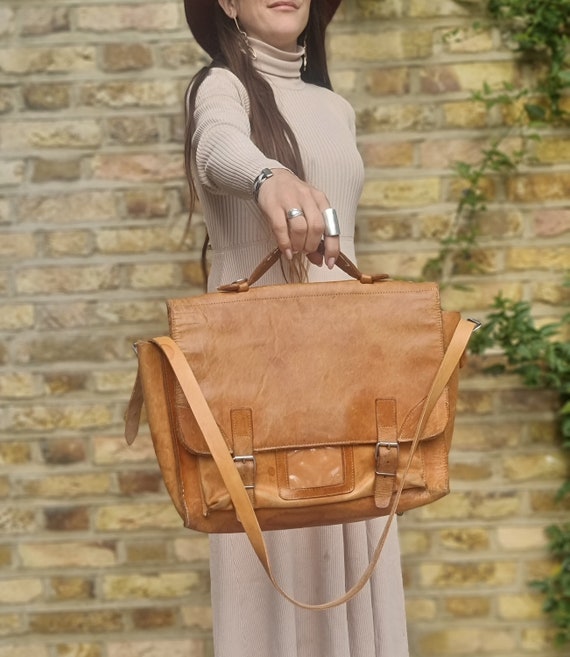This detailed photograph depicts a woman holding out a tan leather satchel towards the viewer. The satchel, which is secured by two leather belt straps with silver buckles, features a fold-over cover, a clear plastic pocket presumably for identification, a shoulder strap draped forward, and a central leather handle by which she is holding it. The woman is dressed in a beige ribbed turtleneck dress that extends to her shins. She accessorizes with silver rings on her right hand's ring and index fingers, and a black and white patterned bracelet on her right wrist. Her long dark brown hair cascades over her shoulders, and her face is visible only up to her upper lip. She stands against a variegated beige and brown brick wall adorned with green vines climbing on one side.